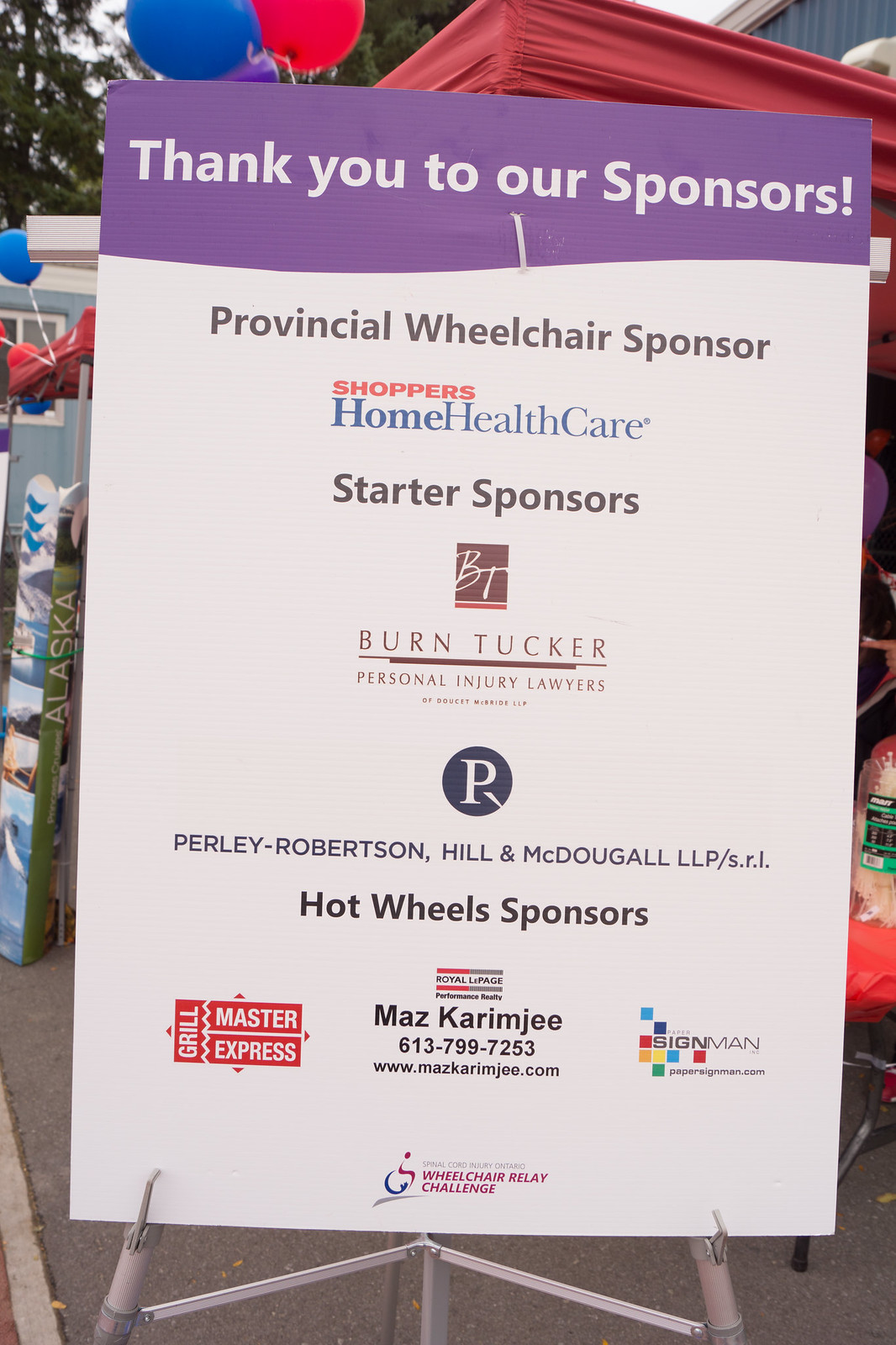The image depicts a tall, rectangular banner mounted on a silver stand on a gray paved sidewalk, slightly tilted to the right. Above the banner, the top of a red tent and a blue and red balloon are visible, hinting at a festive outdoor event. The banner features a wavy purple section at the top with white text that reads "Thank you to our sponsors!" Beneath this, additional information is listed in three sections: 

1. "Provincial Wheelchair Sponsor" followed by "Shoppers Home Health Care" in bold red and blue text.
2. "Starter Sponsors" with several company logos and names symmetrically arranged, including "Burn Tucker Personal Injury Lawyers" and "Perley Robertson, Hill & McDougal LLP."
3. "Hot Wheels Sponsors," listing "Grill Master Express," "Maz Karimji," and "Sign Man." 

At the bottom, the event "Wheelchair Relay Challenge" is mentioned. The overall setting and additional details like a smaller banner with "Alaska" in the background contribute to the lively atmosphere of the event.